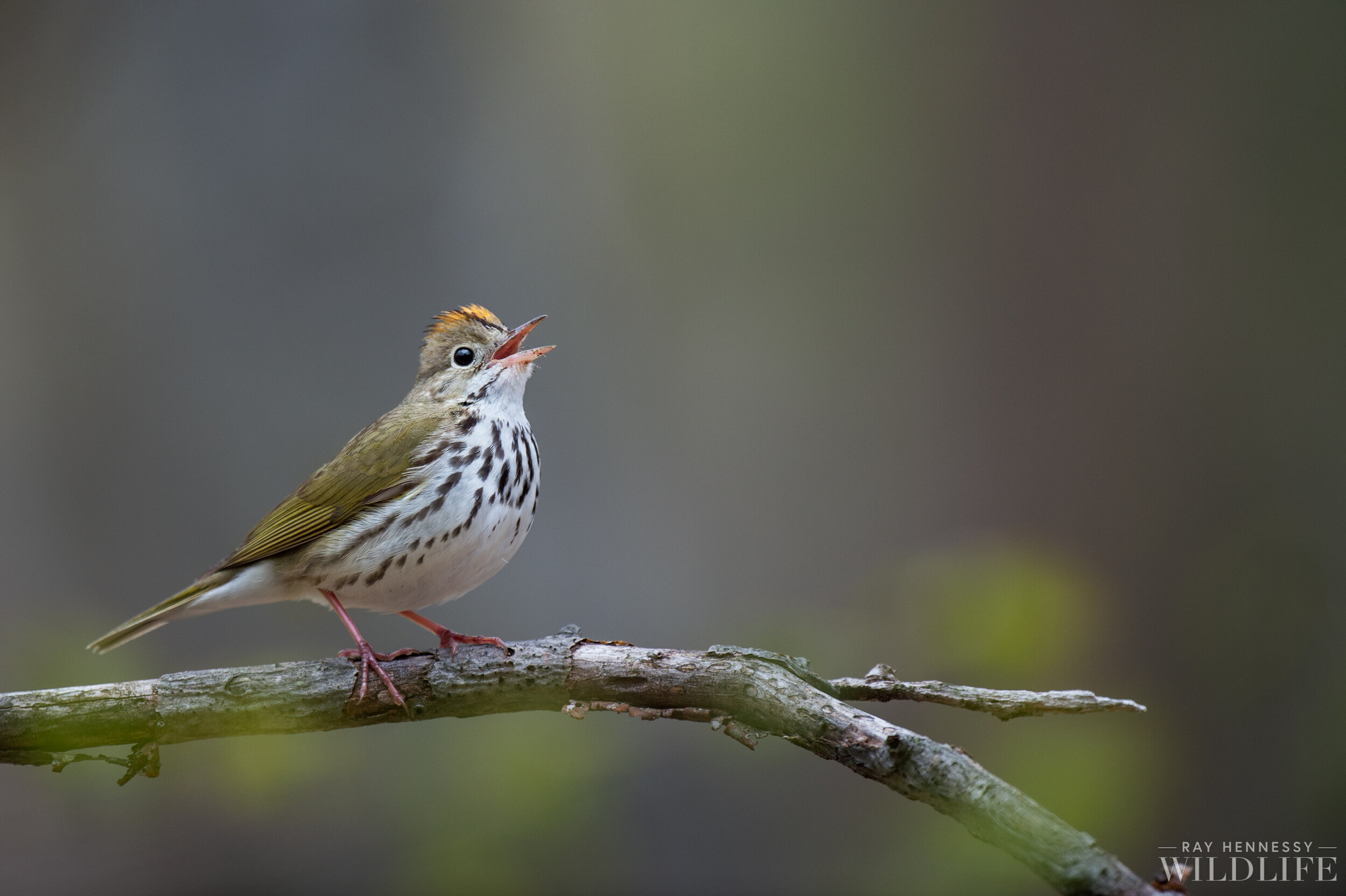The image captures a nature wildlife scene featuring a sparrow-like bird perched on a thin, grayish-tan tree branch. The bird is positioned slightly off-center to the left with an open beak, revealing its peach-colored beak and black eye. Its distinctive features include a small patch of orange feathers on its head and moss green wings. The bird boasts a striking black and white patterned belly, and its red legs grip the branch firmly. The background is a blurred mixture of green, gray, white, and black hues, enhancing the bird's vivid colors. The photographer’s credit, "Ray Hennessy Wildlife," is elegantly inscribed in white in the bottom right corner of the image.